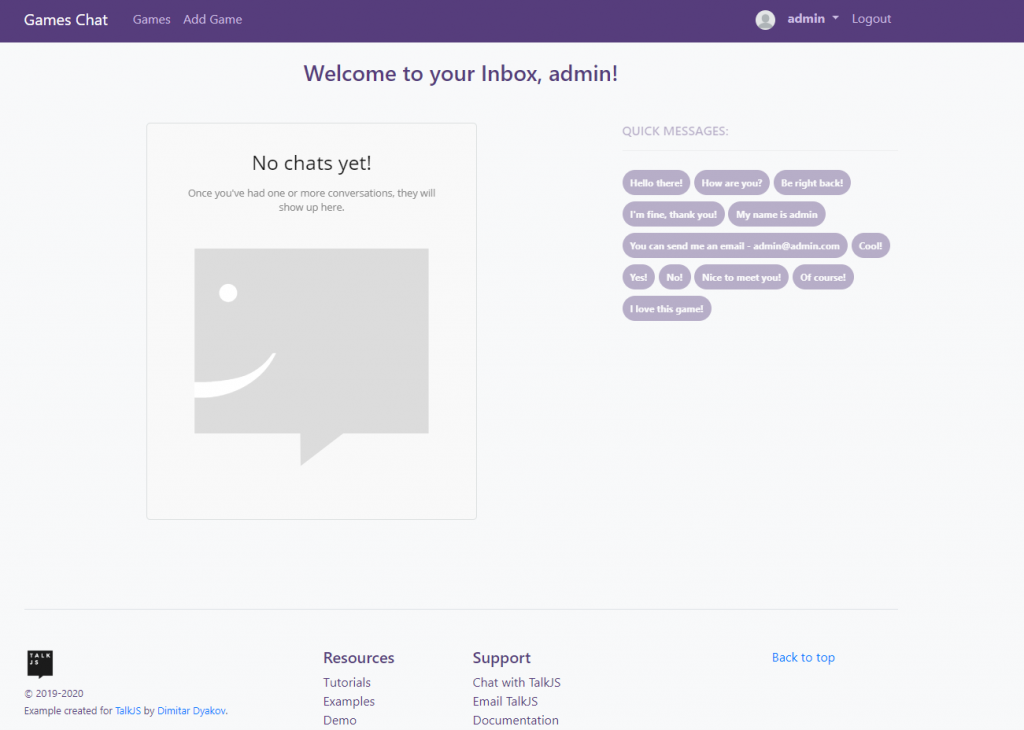**Detailed Caption:**

This image is a screenshot of either a website or an application interface designed for gamers, specifically titled "Gamers Chat." 

- **Header Section:**
  - At the very top, there is a distinctive purple bar running across the screen.
  - On the top left of this bar, the text "Gamers Chat" is displayed prominently.
  - Moving rightwards, the bar features the text "Games" in a slightly smaller font.
  - Further to the right is the text "Add Game."
  - On the top right corner, there is a blank profile picture next to the username "Admin" accompanied by a drop-down arrow for additional options.
  - Adjacent to this is a "Logout" button.

- **Main Section:**
  - Below the header, the main content area of the interface greets the user with the message: "Welcome to your box! Admin!" exclaiming a personalized welcome.
  - Underneath this welcome message, on the left side, there is a rectangular box indicating the absence of chat activity with the text "No Chats Yet."
  - A further explanatory text inside this box reads: "Once you've had one or more conversations, they will show up here."
  - Below this text, there is a smiley face inside a text box.

  - To the right of this rectangular box is another section highlighted in purple titled "Quick Messages."
    - This section contains several preset messages designed to streamline communication:
      - "Hello there."
      - "How are you?"
      - "Be right back."
      - "I'm fine, thank you."
      - "My name is Admin."
      - "You can send me an email at admin@admin.com."
      - "Cool."
      - "Yes."
      - "No."
      - "Nice to meet you."
      - "Of course."
      - "I love this game."

- **Footer Section:**
  - At the bottom of the interface, the footer area is divided into three sections:
    - On the left side, there is a logo alongside a copyright sign, marked "© 2019 and 2020." It also says "Example Created for Talk Us by Dimitar Dyakov."
    - The center section is labeled "Resources," listing "Tutorials," "Example," and "Demo."
    - The right section is dedicated to "Support," offering options to "Chat with Talk.js," "Email Talk.js," and view "Documentation."
    - Finally, at the far right, a blue clickable link reads "Back to Talk."

This detailed description captures all the essential elements of the image, providing a comprehensive overview of the interface's layout and functionality.